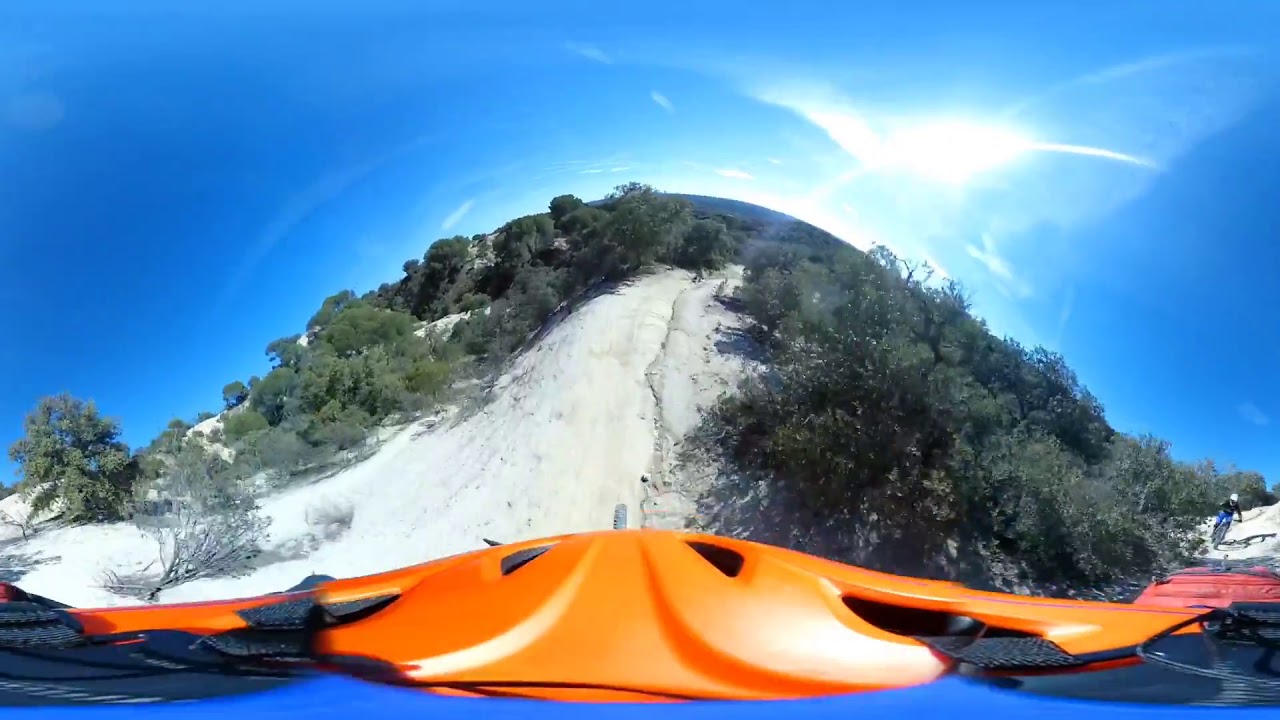The image depicts an outdoor scene featuring a steep, sandy hill framed by abundant green vegetation, including trees and shrubs. Dominating the foreground is the partially visible front of a vehicle, which appears to have an orange and blue color scheme accented with black straps, though only the tip is discernible. The hill's bare central section is prominently sandy, flanked by the greenery on either side. A man on a mountain bike navigates a sandy trail at the lower right corner of the image. Above, the sky is a vibrant blue, punctuated by a bright white flash of sunlight in the top right corner, suggesting a clear, sunny day. The overall setting feels secluded, with the lone biker emphasizing the tranquility of the scene.